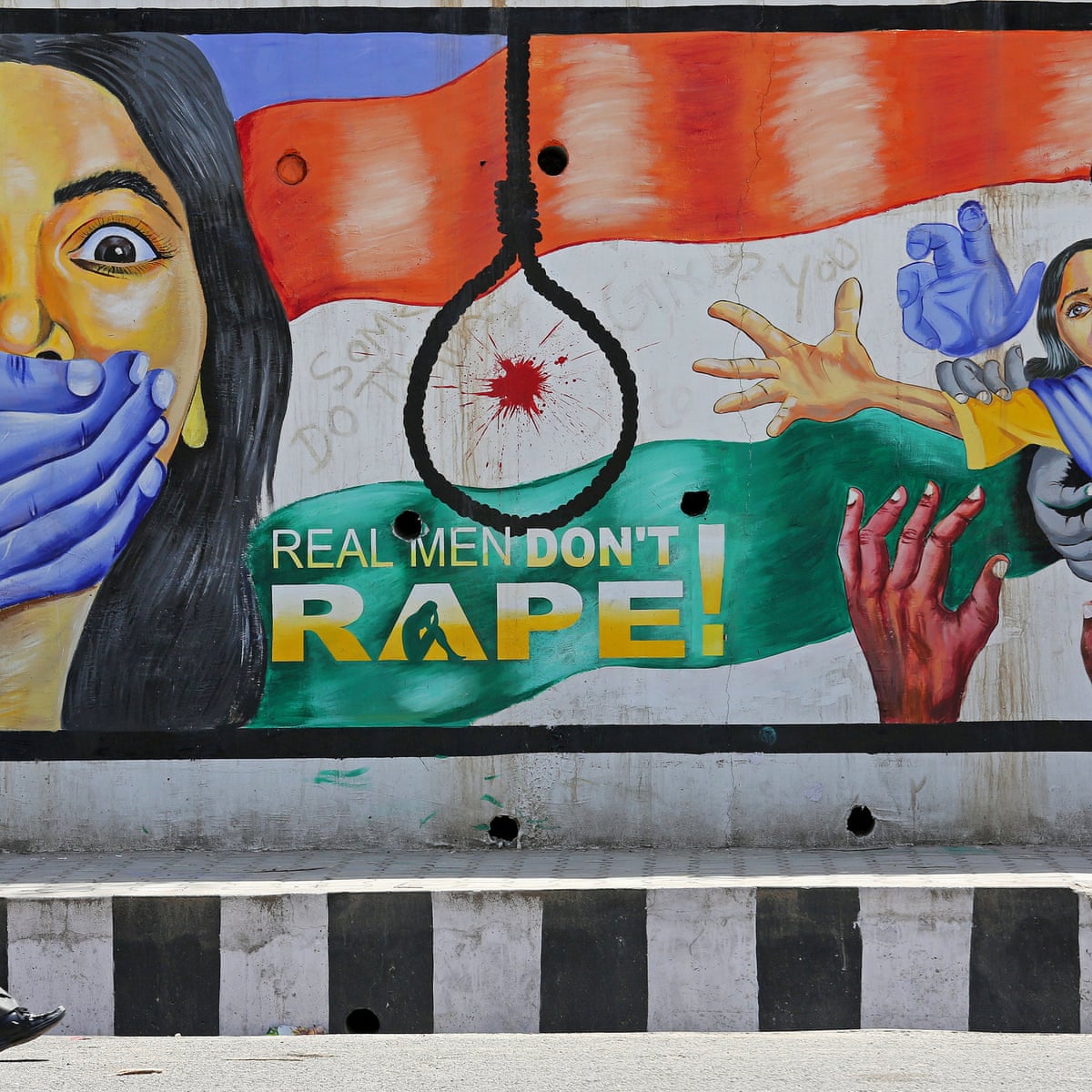The image depicts a poignant and evocative mural on a wall juxtaposed against a sidewalk featuring alternating black and white stripes on its edge. The mural is a powerful statement against sexual violence, with intricate and thought-provoking elements throughout. 

At the bottom of the mural, white and black concrete blocks create a repeating pattern, curving slightly to the right. Above this, a painted flag resembling that of India spans horizontally with orange at the top, white in the middle featuring a blood splatter, and green at the bottom. Encircling the blood splatter in the center white stripe is the silhouette of a noose, symbolizing grim consequences.

The mural features the distressing imagery of abuse: on the left side, a woman with wide-open eyes and a blue hand covering her mouth stands in silent terror. On the right side, a young girl is depicted being grabbed by gray, blue, and red hands, her arm outstretched in a desperate plea for help.

In darker and bolder highlights, swirling lines appear at the very top of the mural, including a red one, a blue one above it, a white one below the red, and a green one stretching horizontally. 

The potent message "Real Men Don't Rape" is written across the mural in prominent yellow and white text. The word "rape" is emphatically displayed in all caps, with the letter “A” containing the haunting silhouette of a person sitting with their head in their hands, possibly crying. This powerful artwork serves as a vivid call to action and an unflinching condemnation of sexual violence.